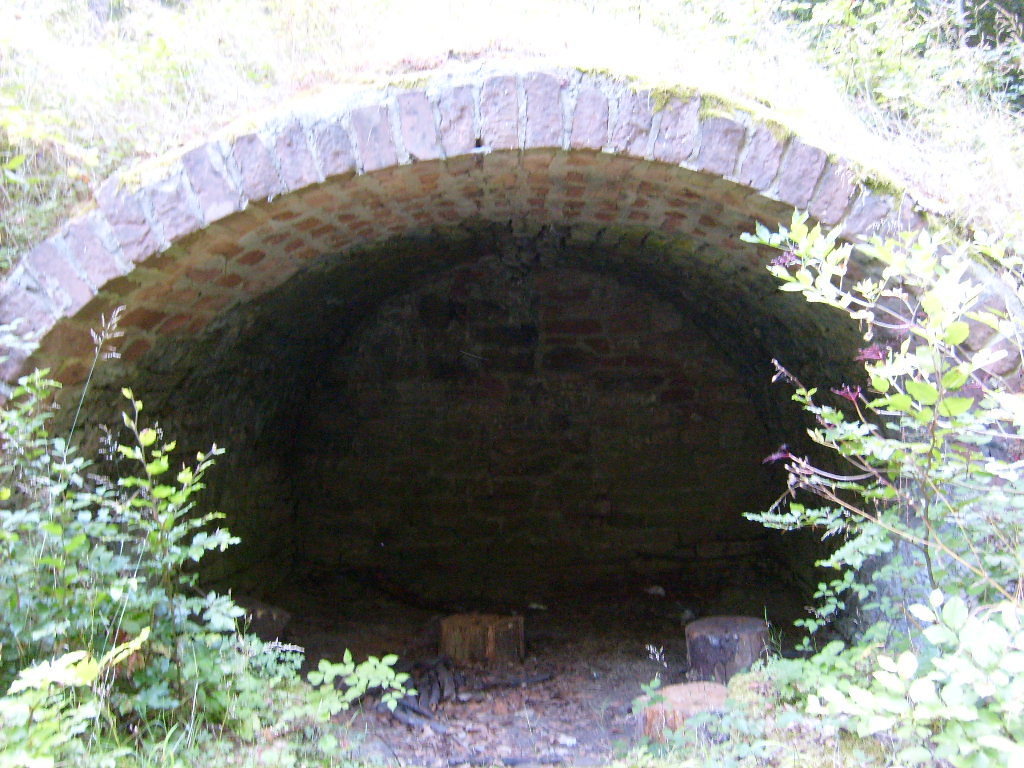The image depicts an outdoor, mid-day setting featuring a rocky, grassy area with various green shrubs and bushes scattered throughout. In the center of the image, there is a brick structure that appears to be built into the side of a grassy hill, resembling a shelter or hideout. This structure features an arched brick entrance that suggests a tunnel or underground room. Inside, the interior is quite dark, but two wooden stumps can be seen, possibly serving as seating arrangements. The brick ceiling reveals a distinct square pattern. The ground leading up to the structure lacks grass, contrasting with the surrounding verdant foliage. Above the arch, the top of the brick structure is adorned with moss and leafy branches that protrude, blending seamlessly with the natural surroundings. The prominent colors in this image include various shades of green, brown, gray, yellow, red, maroon, and white, contributing to the earthy and rustic atmosphere of the setting.